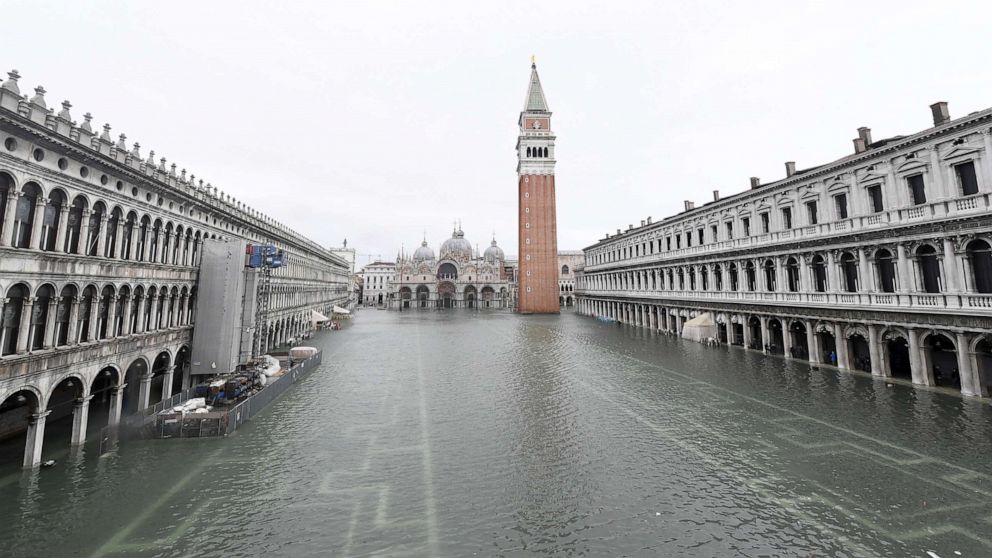The image depicts a flooded canal in an old European-like city, dominated by cloudy, whitish-gray skies. Murky gray water engulfs the area, rising approximately four to five feet off the ground, suggesting recent flooding. In the foreground, a prominent reddish-brown tower with a pointed tip stands out, featuring a white section with small windows near the top. This tower is flanked by tri-level buildings lining both sides of the canal, characterized by gray cement facades with arched window-like structures, possibly bridges, under which boats and barges are moored. The buildings on either side stretch towards the background, where a grand, palace-like structure with domed tops and spires looms, lending an elegant and detailed contrast to the scene. The overall atmosphere is subdued and almost sepia-toned, giving the image a faded, nostalgic feel. Despite the water inundation, no people are visible, perhaps having evacuated to safety.